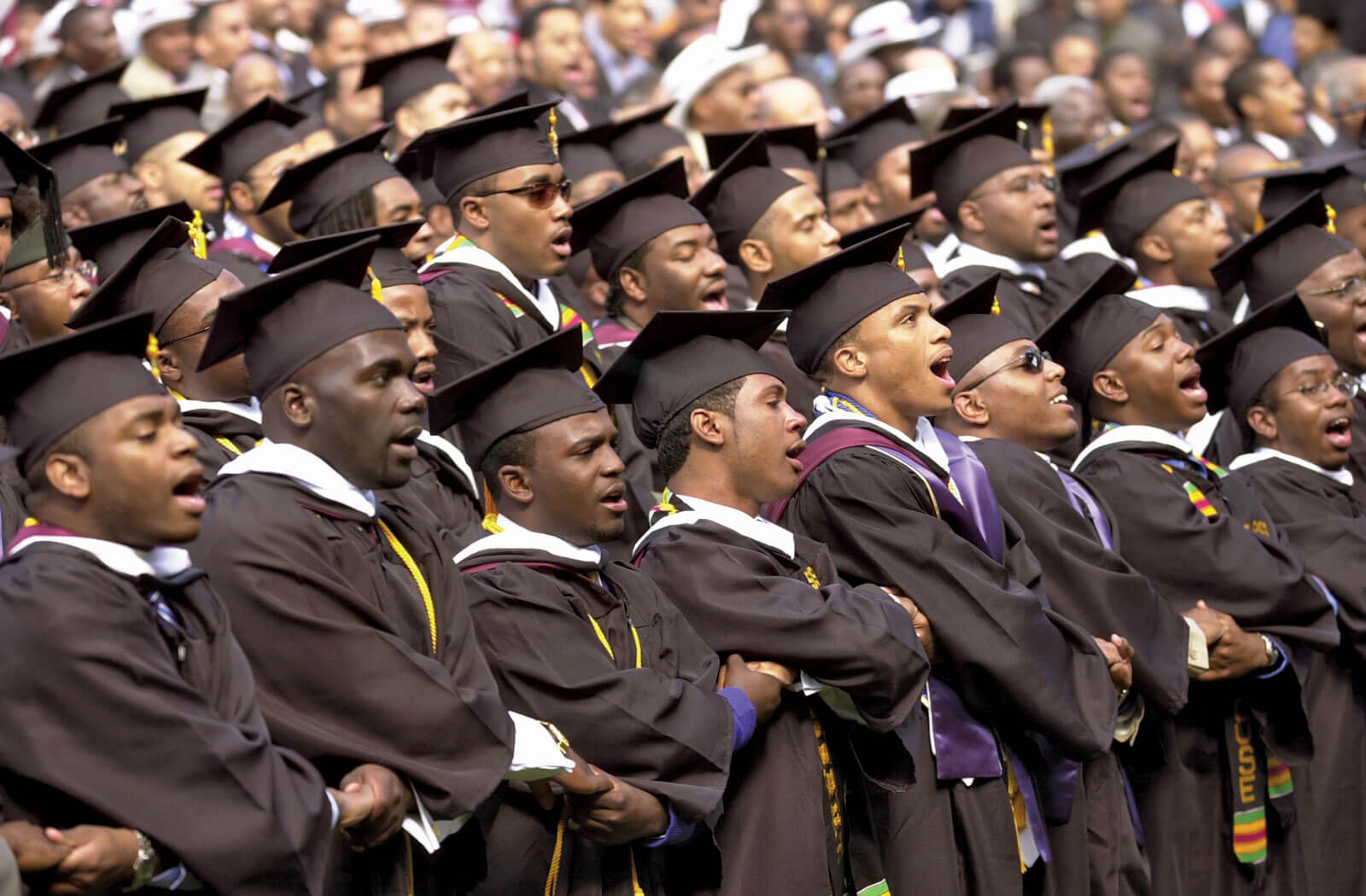This photograph captures a joyful and celebratory scene of a graduation ceremony at a historically black college. The image focuses on a large group of young black men, all dressed in black gowns and caps with their tassels to the left, signifying they have graduated. These graduates form at least four rows and are standing closely together with their arms crossed, holding hands with the person next to them. They are either singing the alma mater, a hymn, or chanting, creating a unified and powerful moment. Some of the graduates have ribbons around their collars, with a few donning purple colors, possibly indicating special honors like valedictorian. The graduates are in sharp focus and somberly yet joyfully celebrate this significant achievement.

In the background, slightly out of focus, stands a crowd of bystanders—likely family members and relatives—who are mostly also black. They are respectfully dressed and some wear different types of hats, distinguishing them from the graduates. The spectators appear to be singing along, contributing to the atmosphere of unity and celebration. Despite the large number of participants, both graduates and attendees, the photograph conveys a sense of connectedness and shared accomplishment within the black community. The scene is illuminated by daylight, further enhancing the vibrancy and warmth of this memorable occasion.